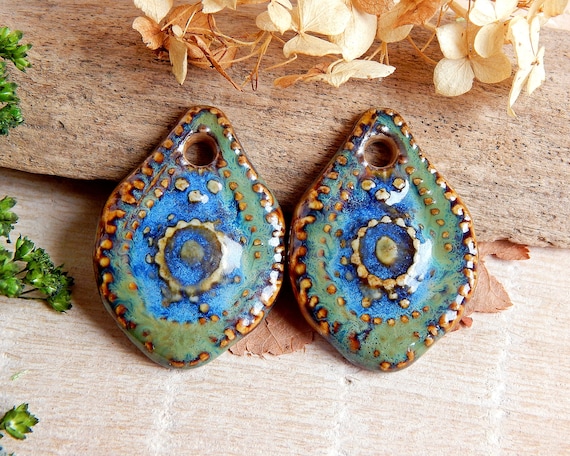In this photo, two intricately designed teardrop-shaped ceramic objects, possibly earrings, rest on a light wooden table. These sculpted items feature a detailed pattern with bluer-green teardrop shapes centered by gold-bordered, circular blue spots, each dominated by a smaller yellow dot. The teardrops are edged with a distinctive golden fringe and have a drilled hole at the top, hinting at their potential use for hanging. Above and around these objects, off-white and blondish dried flowers, along with green leaves, add a delicate natural touch to the composition. The objects share a harmonious yet unique design, making them an intriguing centerpiece on the table.